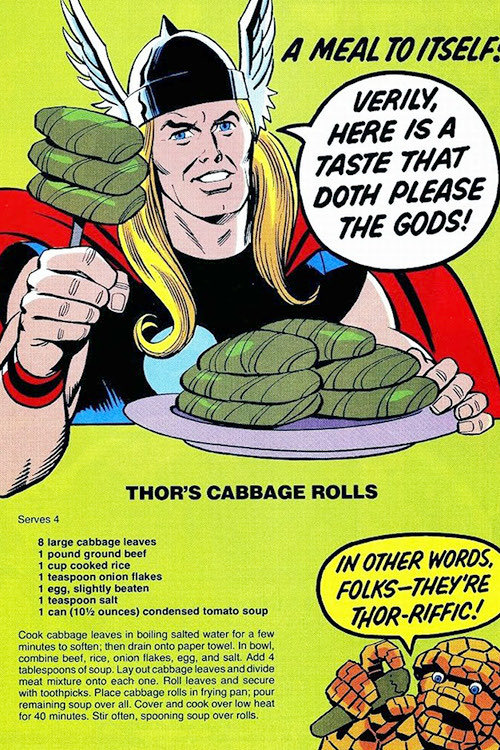This image is a whimsical recipe card with a vibrant lime green background and a vertical rectangular frame. The top half features Thor, the iconic Marvel comic character, resplendent with long blond hair, a metal helmet with winged accents, a black tunic, and a red cape. In dramatic black font, the phrase "A meal to itself" is displayed, accompanied by Thor's speech bubble proclaiming, "Verily, here is a taste that doth please the gods." Thor is holding a plate of cabbage rolls, with three speared on a fork. Below, the header "Thor's Cabbage Rolls" introduces the recipe, detailing ingredients such as eight large cabbage leaves, one pound of ground beef, one cup of cooked rice, one teaspoon of onion flakes, one egg, one teaspoon of salt, and one can of condensed tomato soup. The lower right corner features a smaller image of Ben Grimm (The Thing), captioned with, "In other words, folks, they're Thorific."